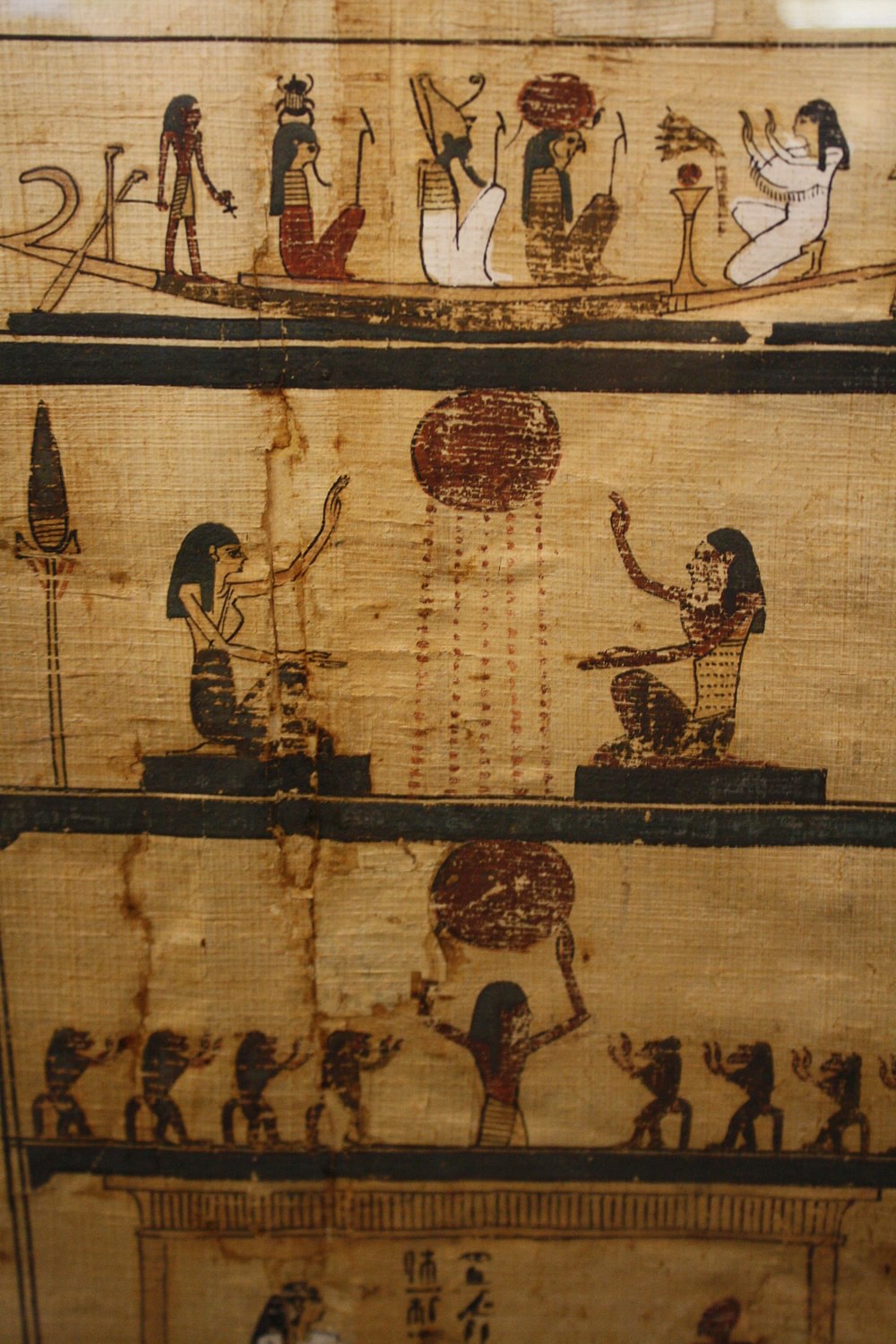This image appears to be a detailed photograph of a rectangular piece of papyrus adorned with intricate Egyptian drawings, segmented into three and a half distinct horizontal scenes. At the top is a depiction of five individuals on a boat or canoe, with four seated towards the right and one standing to the left next to an oar. These figures are adorned in various colors: two in white, two in gold, and one in red. Notably, several of them have objects on their heads, possibly indicating royalty or status, with one woman in particular appearing to bow down to the others.

The second scene portrays two figures seated on either side of a large, circular object emitting rays, reminiscent of the sun or moon. Both figures, one seemingly a woman with black hair and the other possibly a man, have their hands raised, engaged in what suggests a form of worship. Nearby, there is a tall, slender object that could be a corn stalk or a spear.

In the third scene, the circular object is raised above by one figure, while seven smaller figures—potentially people or animals—are positioned around them, three to the right and four to the left, appearing to praise the object. 

The final, partially visible scene at the bottom of the photograph is more ambiguous, showing just the head of a figure, making it difficult to discern their identity or actions. The artistry and arrangement hint at a narrative or ritualistic progression, capturing moments of ancient Egyptian life and beliefs.